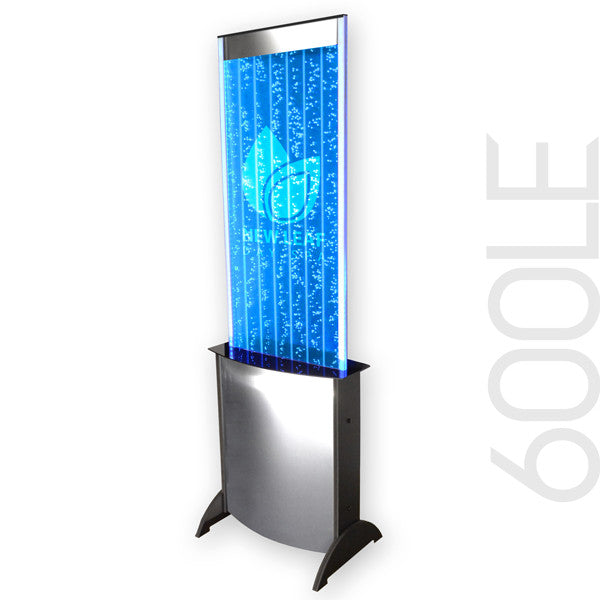The image depicts a sophisticated machine featuring a base made of silver metal, supported by two black legs that may be plastic. Rising from this base is a sleek, black shelf from which a tall, retractable vertical screen emerges. This screen has a unique appearance, with a metallic silver top and a portion projecting a blue image. The image displayed includes white text that reads "new leaf" alongside an illustration of two leaves. The text and design evoke a serene, flowing motion, reminiscent of a modern twist on a lava lamp, suggesting a potential application in virtual reality or high-tech displays typically seen in a retail environment.